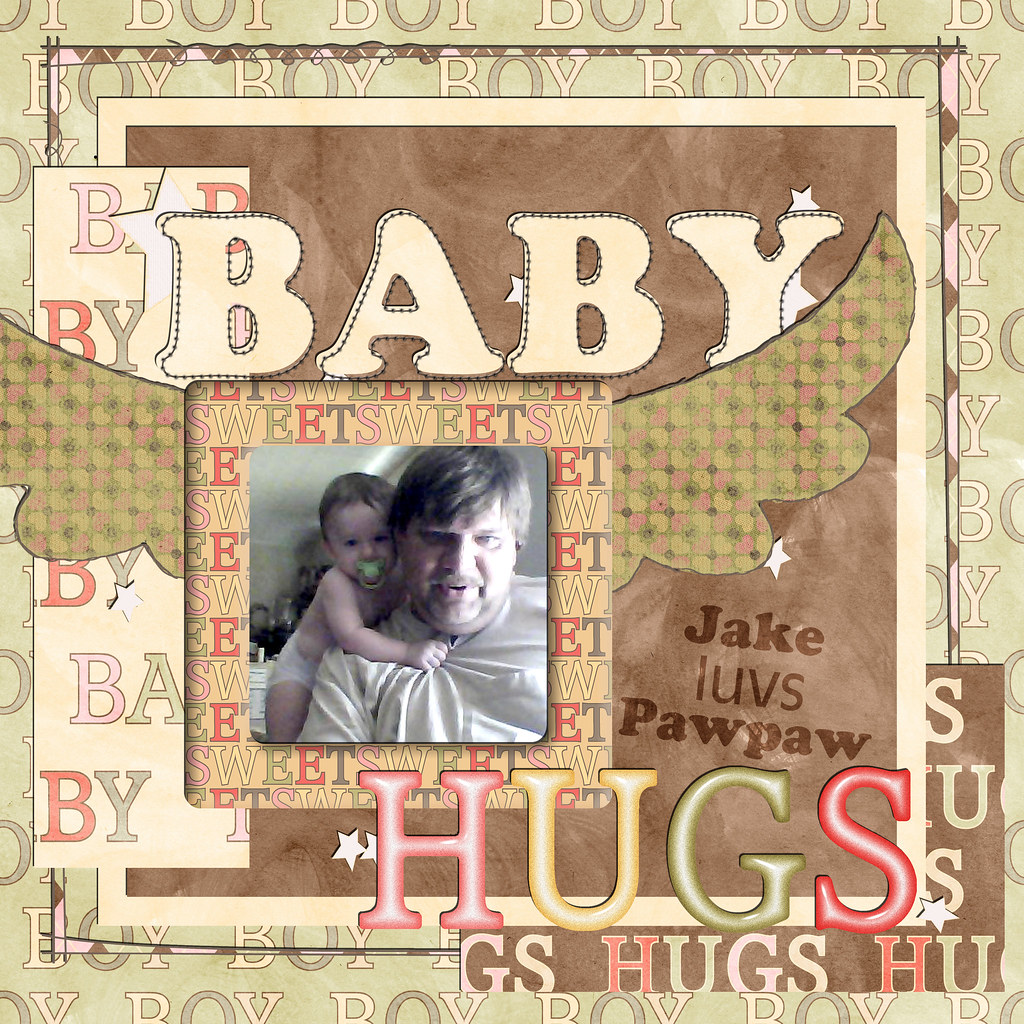In the center of this large square image is a small, framed photograph of a dad and his baby. The dad, wearing a white t-shirt, has short, shaggy brownish-blonde hair and appears to be taking a selfie with his mouth open. Over his right shoulder, his baby, with similar short blondish-brown hair, is wearing only a diaper and has a green pacifier in their mouth. This central photo is framed by text that repeatedly says "sweet" in various colors.

The surrounding border of the image features a textured collage with the word "boy" printed repeatedly in a pattern, alternating between light brown for 'B' and 'Y' and darker brown for 'O.' Above the central photograph, large bubble letters spell out "BABY" in a tan color with a dark brown swirled background. To the right of the photo, text in brown reads "Jake luvs PAWPAW", with "HUGS" below it in large, multicolored letters (pink, yellow, green, red). The overall appearance suggests a mixed-media digital collage, possibly designed to resemble a greeting or thank-you card.